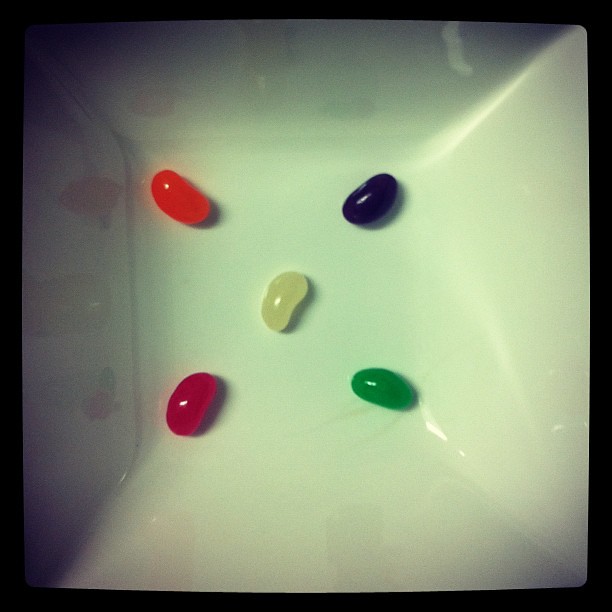The image is a detailed photograph of five jellybeans arranged on a square, white ceramic plate with slightly depressed sides, reminiscent of a shallow bowl. The background of the image is completely black, emphasizing the plate and its contents. The arrangement of the jellybeans mimics the pattern of the number five on a die, with one jellybean in each corner and one in the center. Starting from the top left, the jellybeans are positioned as follows: an orange jellybean in the top left corner, a black jellybean in the top right corner, a red jellybean in the bottom left corner, a green jellybean in the bottom right corner, and a white jellybean in the middle. The perspective is top-down, capturing the details of the reflections and shadows on the smooth surface of the plate. The photograph appears to have a slight darkening filter, adding to the contrast and highlighting the colors of the jellybeans against the stark black background.